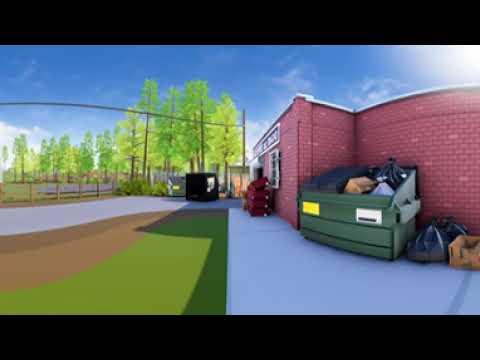This image depicts a computerized scene of a single-story, pinkish-brown brick building with a curved side. Positioned against the wall of the building is a green trash can with a partially open right lid and a closed black left lid. The bin is overflowing with garbage, including a black trash bag, a white trash bag, and a box. Additional trash bags and a box are scattered on the ground next to the container. The building is bordered by a concrete sidewalk and a patch of green grass. On the left side of the frame, tall trees and possibly a fence indicating a park or baseball field can be seen. The sky is a bright blue with some wispy white clouds, suggesting it is a sunny day.